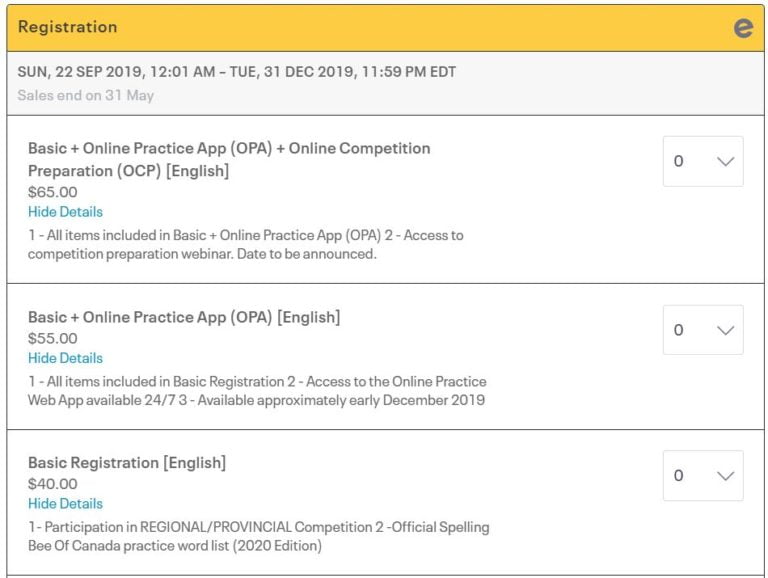**Detailed Event Registration Information**

**Registration for Competition**

**Dates:**  
- Sunday, September 22, 2019, 12:01 a.m. through Tuesday, December 31, 2019, 11:59 p.m. (Eastern Daylight Time)
- Sales end on May 31

**Options and Pricing:**

1. **Basic and Online Practice App (OPA) + Online Competition Preparation (OCP)**  
   - **Price:** $65  
   - **Includes:**  
     - All items included in the Basic and Online Practice App (OPA)
     - Access to competition preparation webinar (date to be announced)

2. **Basic and Online Practice App (OPA) in English**  
   - **Price:** $55  
   - **Includes:**  
     - All items included in Basic Registration
     - Access to the online practice web app available 24/7 (approximately available in early December)
     - Does not include online competition preparation

3. **Basic Registration**  
   - **Price:** $40  
   - **Includes:**  
     - Participation in regional/provincial competition
     - Official Spelling Bee of Canada practice word list (from the 2020 edition)

**Note:** The registration displayed prominently with a yellow box at the top, with a white background for the remaining details.